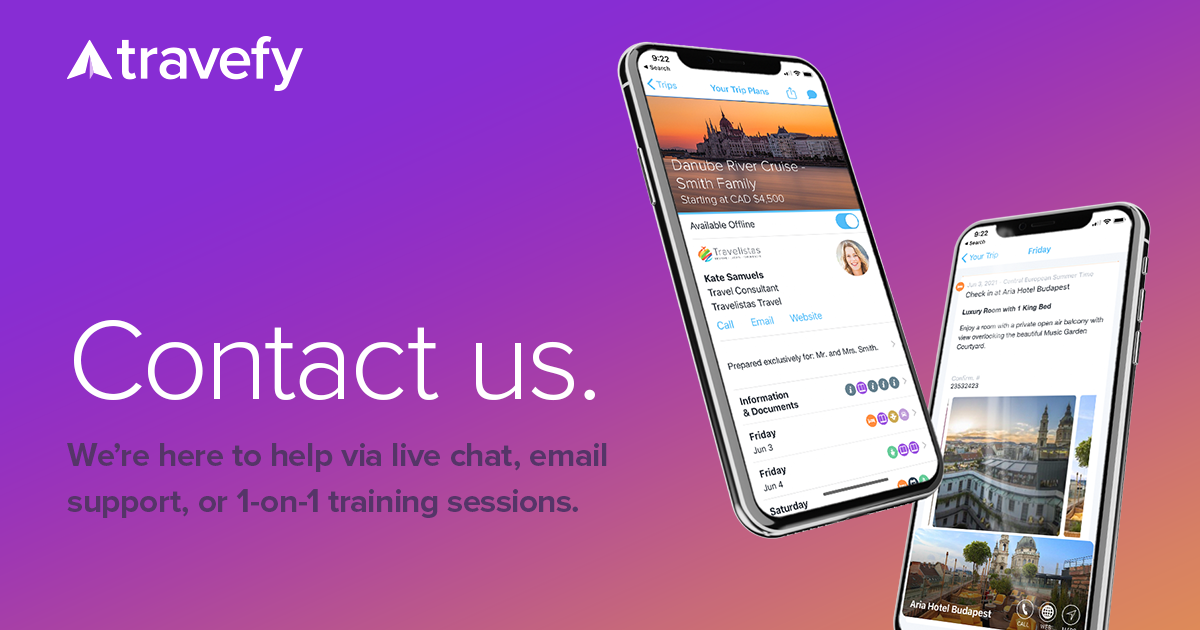*Travify Advertisement*

The upper left corner of the advertisement features the Travify logo, which resembles a paper airplane, positioned prominently against a purple background that fades into a pinkish-orange hue reminiscent of a sunset. The bottom left corner of the ad contains the text "Contact Us" in large white letters. Beneath it, in smaller dark grey text, it reads: "We're here to help via live chat, email support, or one-on-one training sessions."

To the right side of the advertisement, two cell phones are displayed. One phone showcases a planned vacation for a Danube River cruise tailored for the Smith family, with a starting price of CAD $4,500. The itinerary is prepared exclusively by Kate Samuels, a blonde travel consultant from Travelista.

The detailed itinerary includes costs and essential travel information, such as departure dates and daily activities. The rightmost phone displays images and details of the Hotel Budapest, where the Smith family will stay. The hotel features a luxury room with one king bed, and additional photos highlight the hotel's beautiful exterior, complemented by a picturesque sky and surrounding trees.